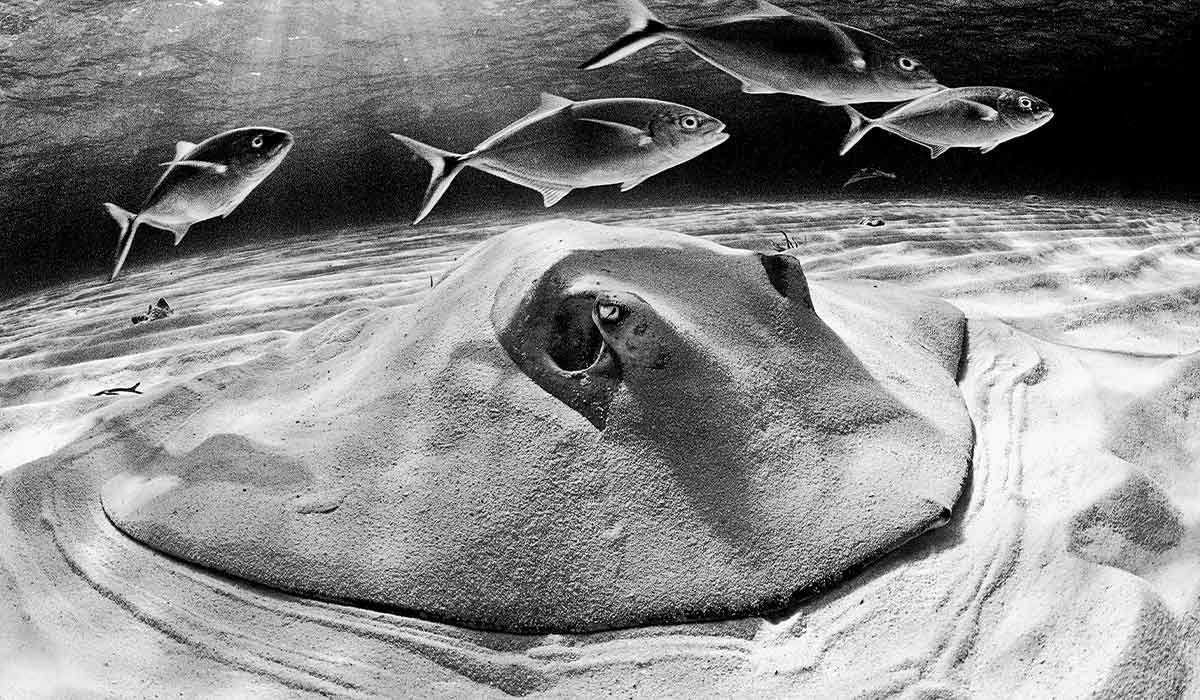In this detailed black-and-white artwork, we dive into a striking underwater scene. At the top, rays of sunlight penetrate the water surface, illuminating the ocean depths with dramatic beams. Four small fish swim together near the surface, their movements captured in delicate yet vivid detail. Their presence provides a stark contrast to the ocean floor below, which is dominated by a stingray. The stingray is almost entirely camouflaged, dusted and coated with sand, blending seamlessly into the textured seabed. One of its eyes is visible, peering menacingly up towards the unsuspecting fish. The artwork, meticulously detailed in shades of black, white, and gray, creates a captivating portrayal of a hidden predator lurking in its natural habitat, poised for an ambush.